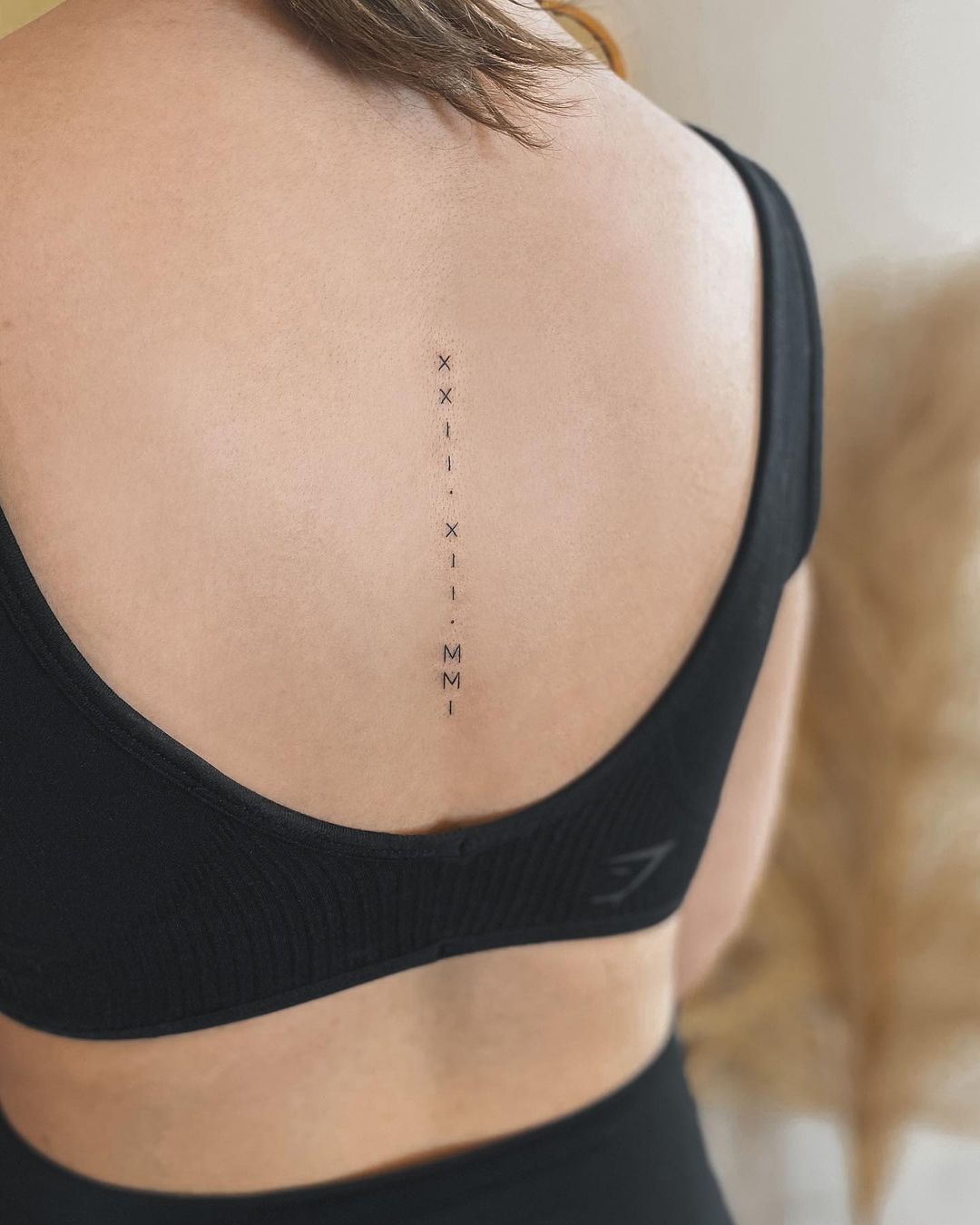The image depicts the back of a light-skinned woman with brown hair just visible at the top of the frame. She is facing away from the camera, wearing a black sports bra or low-cut crop top and black bottoms, which could be spandex shorts or leggings, though the image is cut off around her waist. Prominently displayed down the center of her spine is a vertically aligned tattoo, featuring the Roman numerals "XXII.XII.MMI," likely representing the date December 22, 2001. The background is blurred, with a light grayish-tan hue and a hint of a golden-brown pompous bush or decorative item to the right. The overall scene is slightly out of focus, emphasizing the clarity of her tattoo and athletic attire.